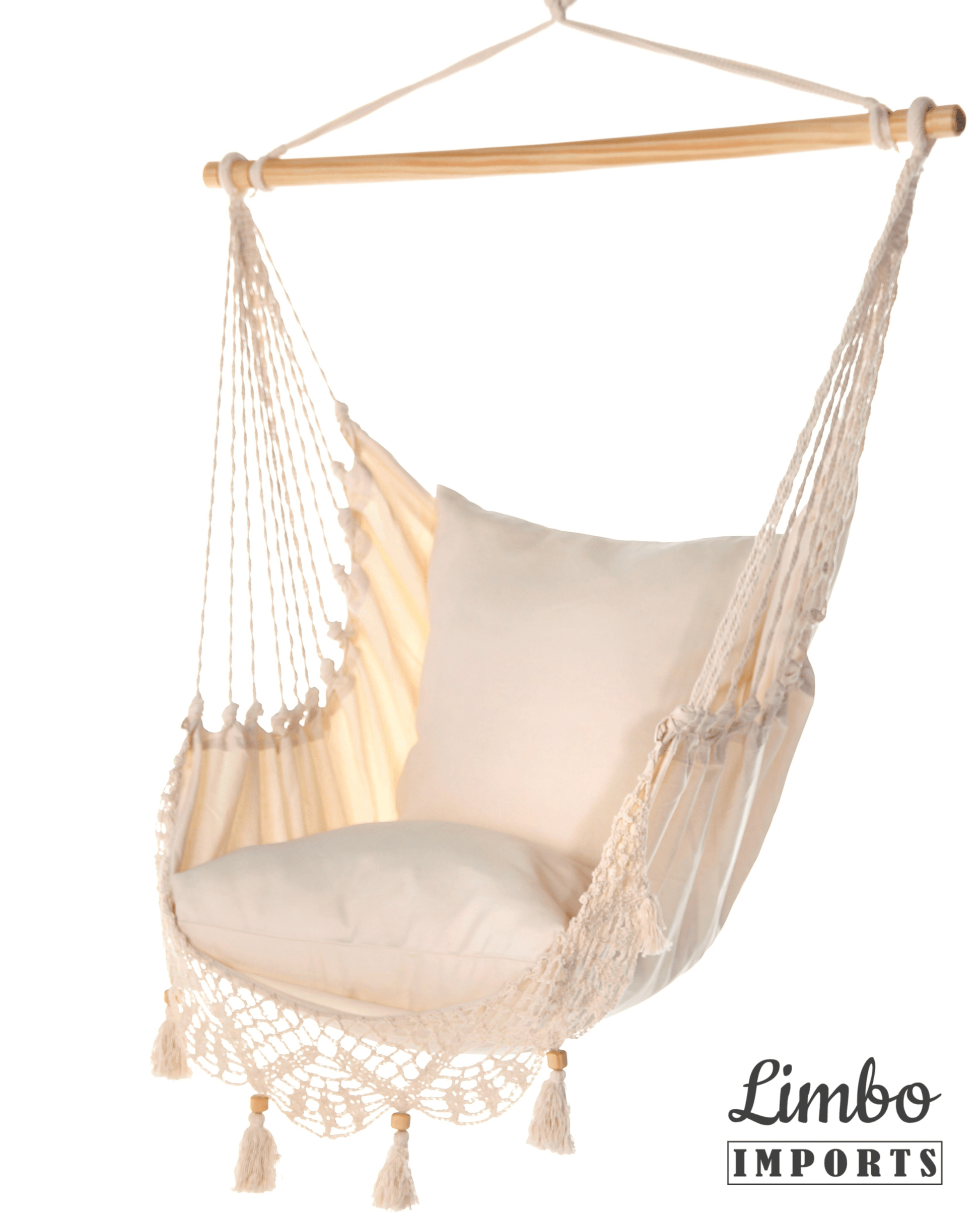The image showcases a hanging hammock chair prominently featured against a neutral background. At the bottom of the image, the branding "Limbo Imports" is displayed, with "Limbo" in cursive and "Imports" in a printed typeface. The chair itself consists of a cream-colored fabric seat supported by multiple small ropes extending from a sturdy natural wooden dowel. The structure above the dowel forms a triangular shape with the rope, enabling the chair to be hung securely. Within the hammock, there are two white pillows for added comfort, one positioned upright and the other laying down. The chair’s front features crocheted detailing, from which hang four white tassels, each adorned with a wooden bead. The overall appearance of the chair is cohesive in off-white tones, enhancing its elegant and simple design.